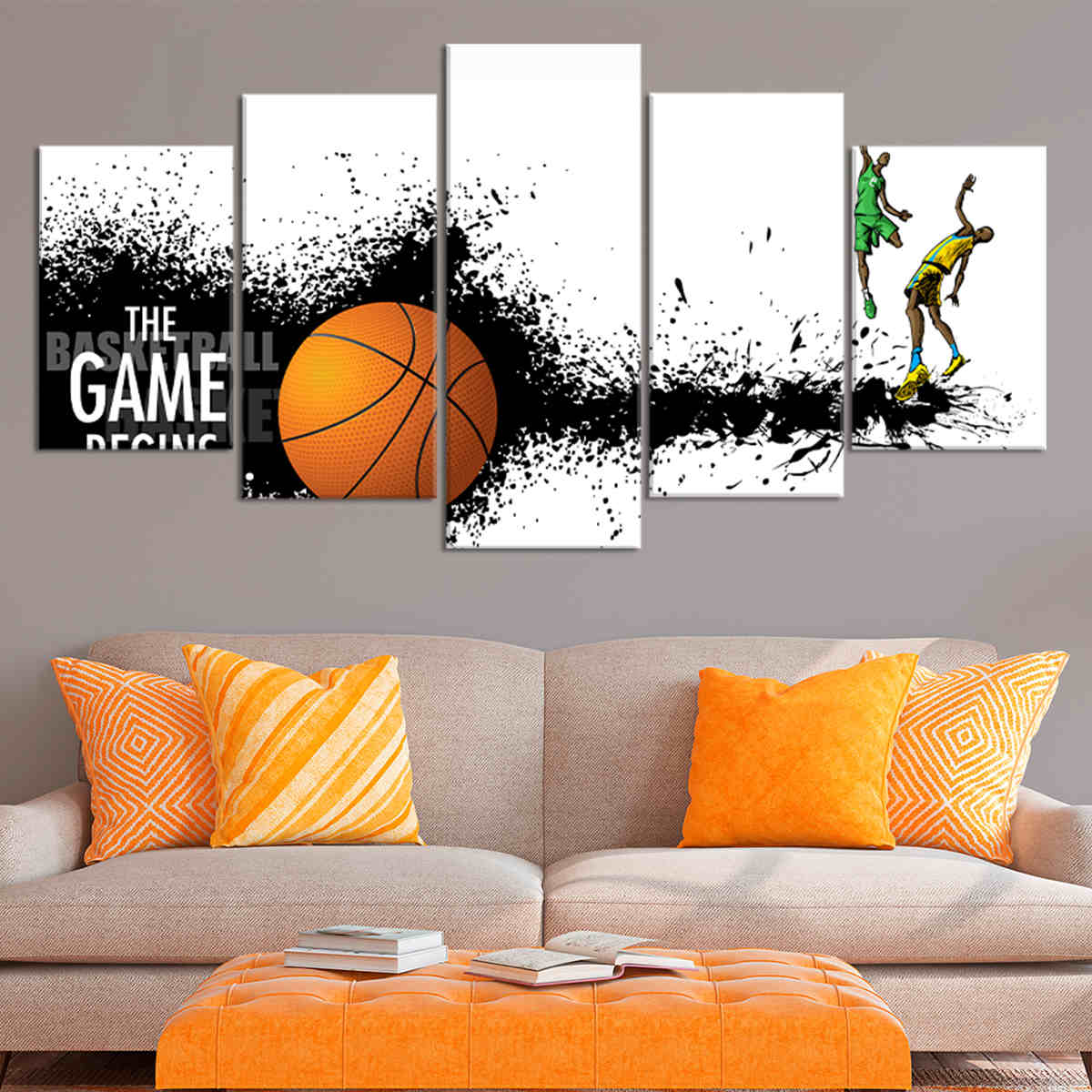The photograph captures a modern living room with a gray wall as its backdrop. Central to the image is a light beige two-seater loveseat adorned with orange and yellow throw pillows, two on each side. In front of the loveseat is an orange tufted ottoman, on top of which lie three books, one open as if someone were in the middle of reading it. Dominating the wall above the loveseat is a striking piece of basketball-themed artwork composed of five rectangular panels arranged in a horizontal line. The first panel features the words "The Game Begins" in black and white. The second and third panels display an orange basketball that matches the colors of the ottoman and the throw pillows. The fourth panel shows a white background speckled with black dots. The final panel captures two basketball players jumping mid-air, completing the energetic and cohesive artwork that ties the room’s color scheme and theme together seamlessly.